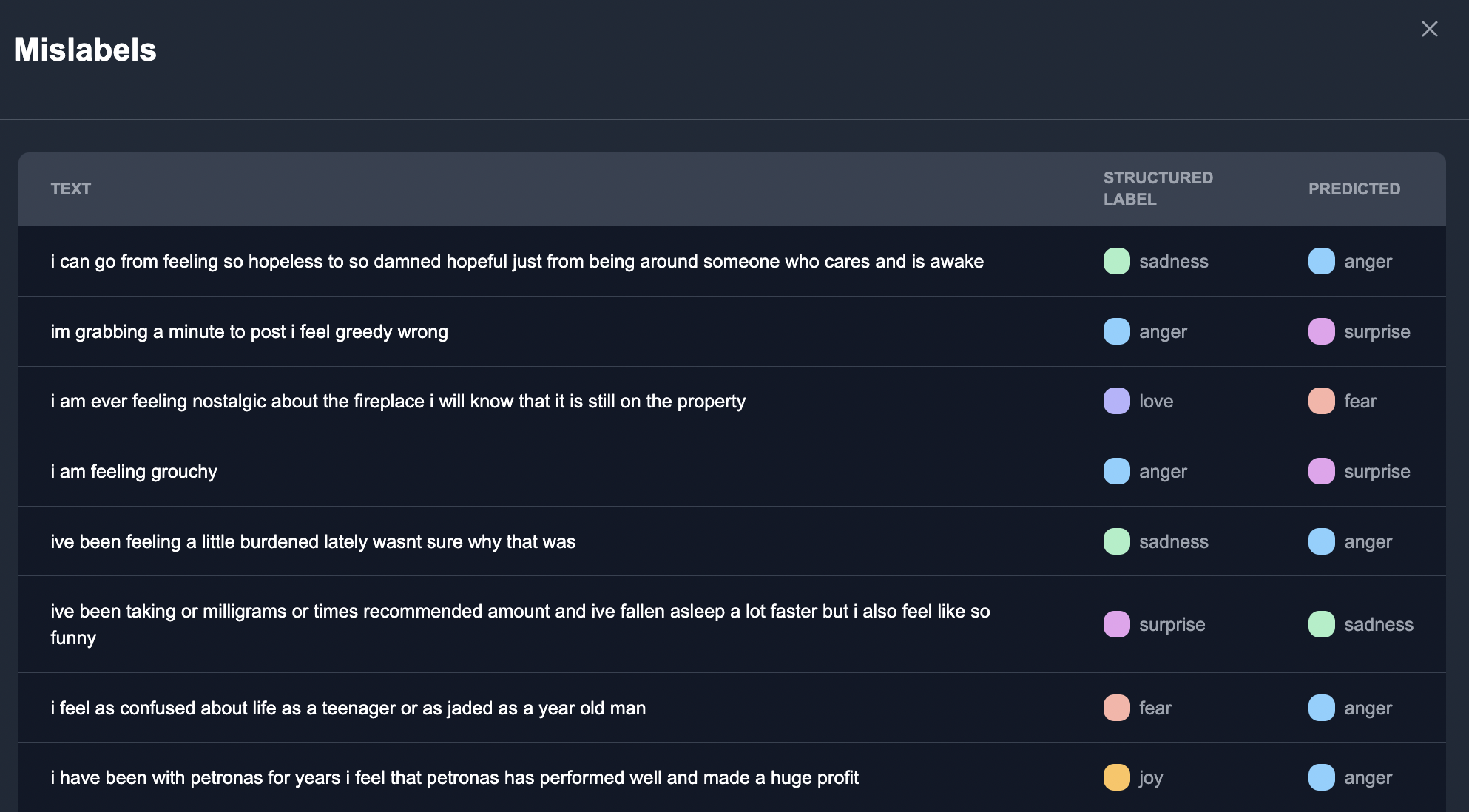**Caption:**
In this image of a computer screen titled "Mislabels," displayed in white text in the upper left-hand corner, the background is predominantly black. Overlaid on the image are various statements and questions illustrating the fluctuations of human emotions. Each sentiment or utterance is paired with structured and predicted emotional labels, demonstrating a comparison between intended and perceived emotions.

The statements include:

1. "I can go from feeling so happy to so damn hopeless just from being around someone who cares and is awake." - Structured Label: Sadness; Predicted Label: Anger.
2. "I'm grabbing a minute to post. I feel greeted, I think it says greedy." - Structured Label: Anger; Predicted Label: Surprise.
3. "I am never feeling nostalgic about the fireplace. I know that it is still on the property." - Structured Label: Love; Predicted Label: Fear.
4. "I am feeling grouchy." - Structured Label: Anger; Predicted Label: Surprise.
5. "I've been feeling a little burdened lately and wasn't sure why." - Structured Label: Sadness; Predicted Label: Anger.
6. "I've been taking milligrams or times the recommended amount and have fallen asleep a lot faster, but also feel strange." - Structured Label: Surprise; Predicted Label: Sadness.
7. "I feel as confused about life as a teenager or as jaded as an older man." - Structured Label: Fear; Predicted Label: Anger.
8. "I have been with patrons for years. I feel that Patronus has performed well and made huge profits." - Structured Label: Joy; Predicted Label: Anger.

The emotions such as sadness, anger, and the feelings are represented by dots of varying colors, including green, blue, purple, pink, gold, and yellow, adding visual differentiation to the predicted emotional states. This sophisticated visualization demonstrates the complexity and variability in recognizing and interpreting human emotions through computational analysis.